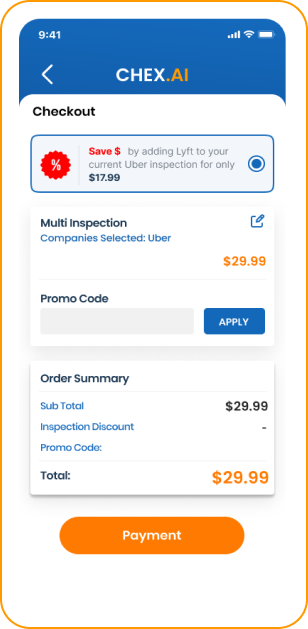This image is a detailed screenshot of a mobile device's portrait mode, framed with a distinct, curved orange border that mimics the shape of the phone screen. There's a thin white border between the screenshot and the orange frame. 

At the very top left of the screenshot, the time is displayed as 9:41, accompanied by full cellular reception, Wi-Fi signal, and battery icons on the right side. Just below this, within a blue header, white text reads "checks.ai" with the ".ai" portion in orange. A back button labeled "Checkout" is positioned to the left.

The main section of the screenshot features a blue box bordered in red, containing bold text that proclaims: "Save money by adding Lyft to your current Uber inspection for only $17.99." A blue radio button, indicating selection, is situated to the right of this text. To the left, a red, percentage-symbol certificate icon is visible.

Below this, the text states, "Multi-inspection company selected Uber for $29.99," followed by a blue edit icon on the right. Beneath this, there is a promo code entry field labeled "Promo Code," accompanied by an "Apply" button. The order summary lists the total as $29.99, culminating in an orange "Payment" button at the bottom.